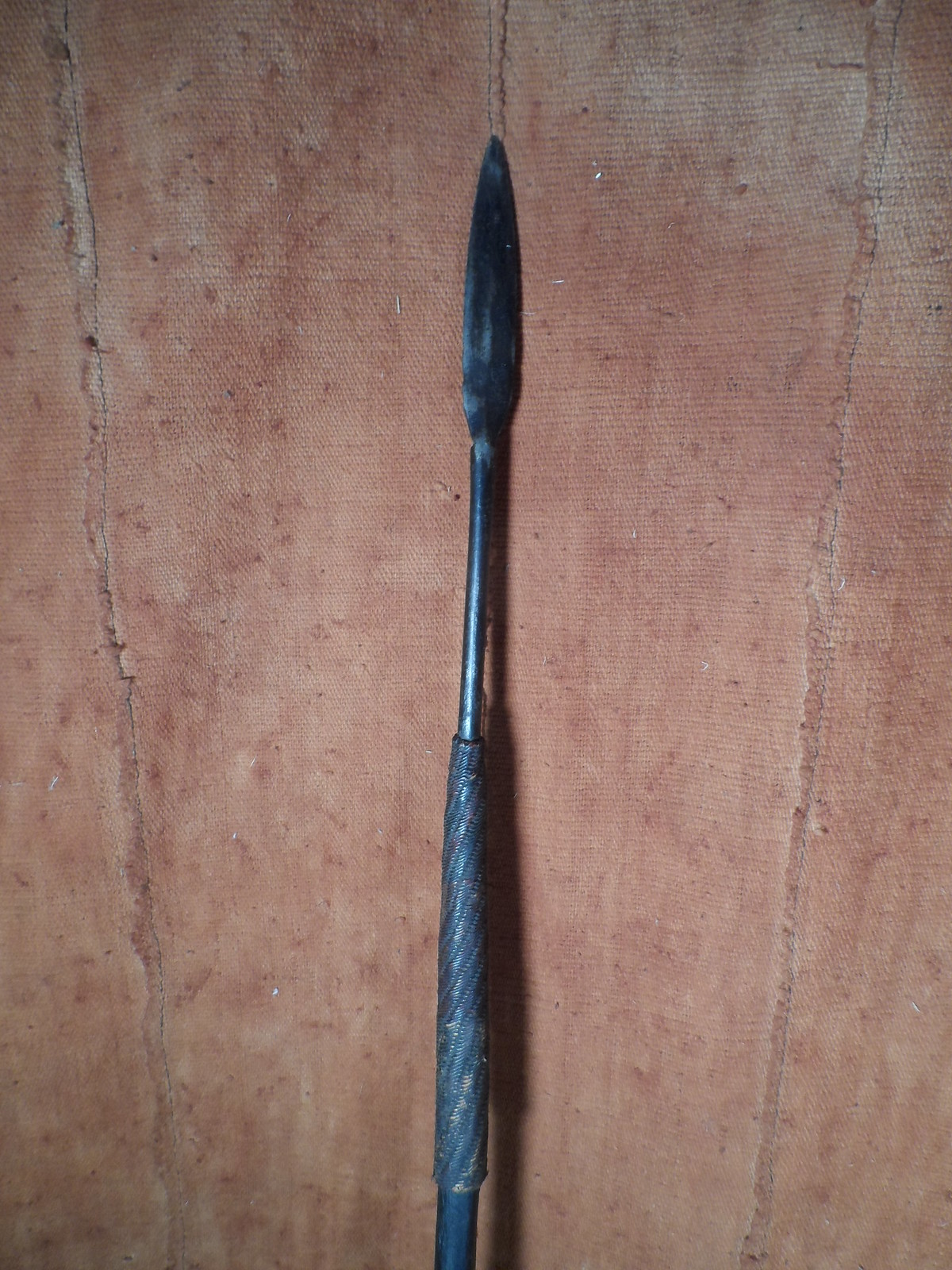The photograph showcases a spear with an iron tip set against a fabric backdrop. The spear, prominently positioned in the center, features a dark gray, aged, and well-used metal handle with a rugged rubber grip near the lower end. Its tip is blunt, tapering to a rounded point reminiscent of a feather's outline, suggesting it has seen significant use. The background fabric, while originally white, is heavily stained with faded red blotches, giving it a distressed, rust-like appearance. The fabric, coarsely woven and vertical in its seam placements, stretches like a curtain across the image. The scene is lit from the left side, casting sharp shadows to the right of the spear, emphasizing the texture and wear of both the spear and the fabric.